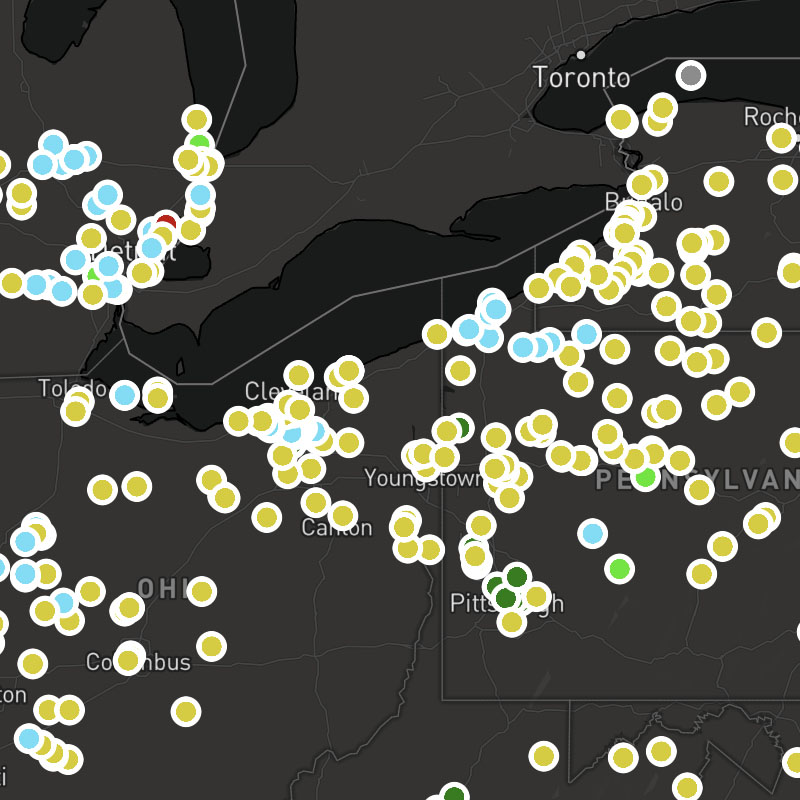This image is a vertical rectangle screenshot of a website displaying a dark gray map, accentuated with varying shades of black representing bodies of water. The map features several points of interest marked by colored dots. At the top right corner of the map is the label "Toronto," followed by "Buffalo" as you trace downward. To the middle left is the region labeled "Pennsylvania," with "Pittsburgh" prominently marked. Just above Pittsburgh, the map indicates "Youngstown." 

The left side of the map highlights the state of Ohio. Here, "Toledo" is positioned to the far left, with "Cleveland" slightly to the right and near the top of the state. Moving further right and downwards, "Canton" is marked, and below that to the left, we see "Columbus." 

Various points of interest are scattered throughout the map, denoted by colored dots which include light blue, yellow, green, and a singular red dot, each representing different locations or landmarks across the mapped area.